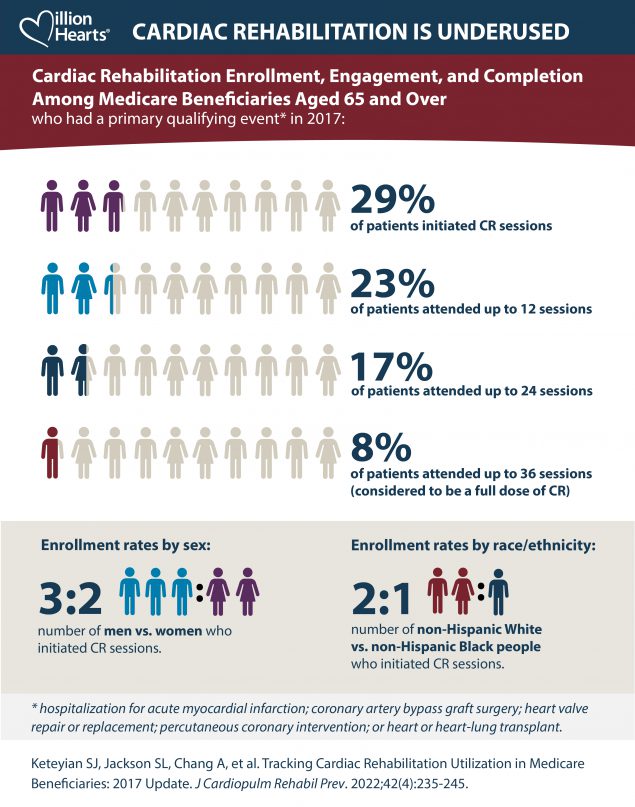This detailed informational poster highlights the underuse of cardiac rehabilitation among Medicare beneficiaries aged 65 and older who had a primary qualifying event in 2017. 

At the top of the poster, a blue rectangle banner with white text announces, "Million Hearts: Cardiac Rehabilitation is Underused." Just below, a maroon banner with white font states, "Cardiac Rehabilitation Enrollment, Engagement, and Completion among Medicare Beneficiaries Age 65 and Over who had a Primary Qualifying Event in 2017."

The main section of the poster consists of four rows of stick figures, conveying different stages of cardiac rehabilitation engagement with the following statistics:
- The first row has approximately 10 figures, with the first three colored purple, and the remaining in white. Blue text next to this row reads, "29% of Patients Initiated CR Sessions."
- The second row also shows around 10 figures, with two and a half colored turquoise blue and the rest white. Beside this row, blue text indicates, "23% of Patients Attended up to 12 Sessions."
- The third row depicts about 10 figures as well, with one and a half figures in green and the rest in white. The adjacent blue text states, "17% of Patients Attended up to 24 Sessions."
- The fourth row features roughly 10 figures, with only one colored maroon and the rest white. Blue text next to it notes, "8% of Patients Attended up to 36 Sessions," which is considered a full dose of cardiac rehabilitation.

Below these rows, a small gray banner highlights enrollment rates by sex and race/ethnicity. This includes a 3:2 ratio (depicted by three blue male figures and two female figures) and a 2:1 ratio (represented by two red figures and one blue figure) respectively. 

At the bottom, small blue text provides the source of the information.

This poster effectively combines vibrant graphics and concise data to emphasize the critical issue of cardiac rehabilitation underuse among the elderly Medicare population.